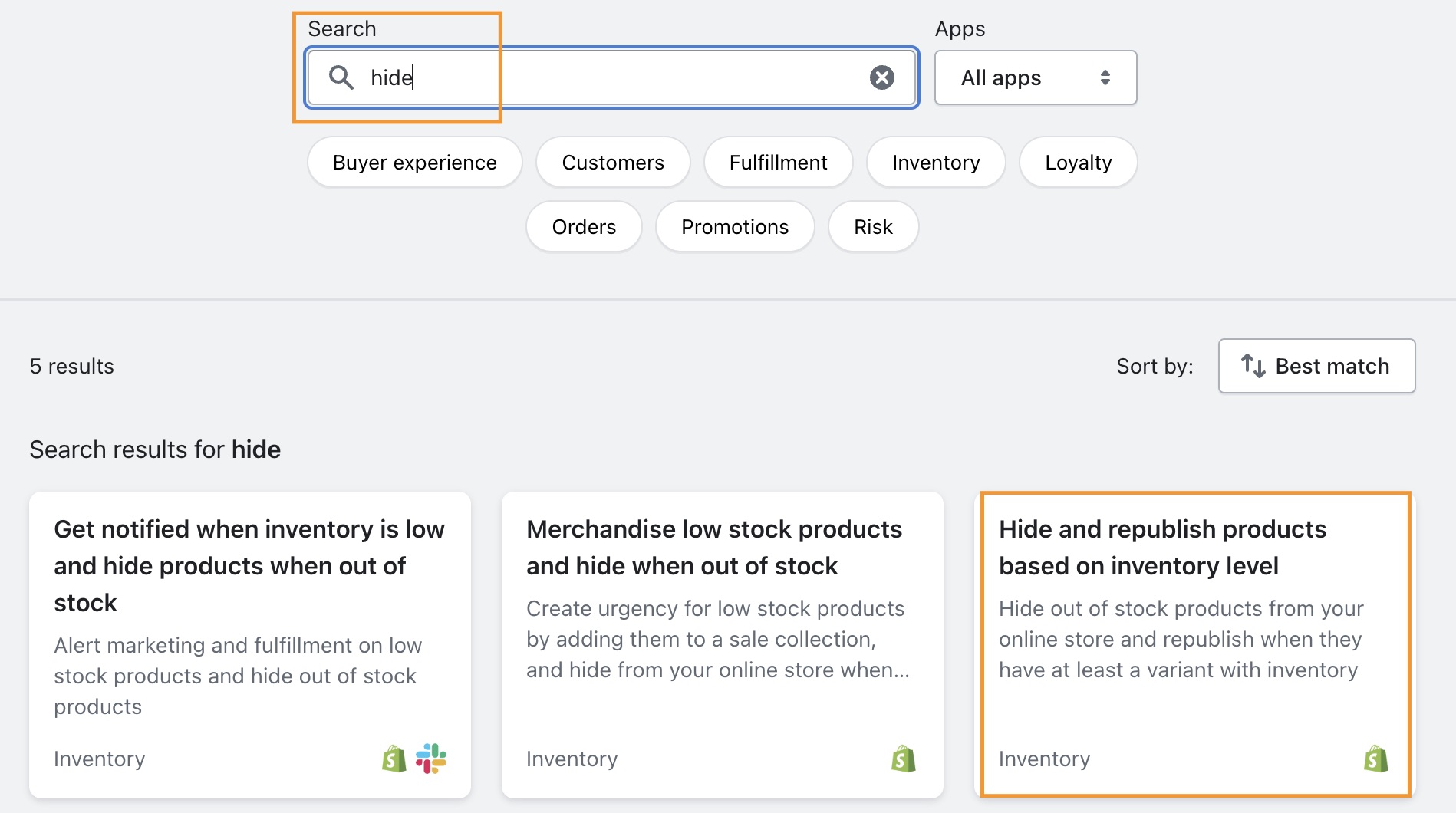This is a screenshot of a user interface showing a search feature. The window has a greenish or grayish hue. At the very top, the word "Search" is prominently displayed, followed by a white search bar where users can input their queries. To the right of this is a dropdown menu allowing users to search within specific apps or categories. 

Below the search bar, a series of tags can be seen, including options like "Our Experience," "Customers," "Fulfillment," "Inventory," "Loyalty," "Orders," "Promotions," and "Risk," providing quick filter options for the search. 

At the bottom of the screen, a message indicates there are five search results for the term "hide," which was entered into the search bar. The search results are displayed in three rectangular boxes arranged horizontally from left to right.